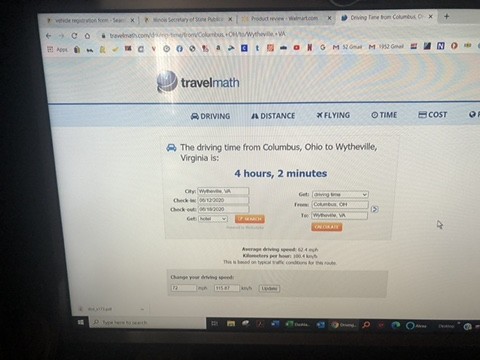This image is a photograph of a computer screen displaying a website screenshot from Travel Math. The background is black, while the main screenshot is white with blue trimming. At the top of the screen, there is a blue banner featuring a small globe icon beside the words "Travel Math." To the right are various labeled categories, indicated by icons and text: a car with "Driving," people with "Distance," an airplane with "Flying," a clock with "Time," and a square block with "Cost." Below this banner, a car icon precedes the text stating, "The driving time from Columbus, Ohio to Wytheville, Virginia is four hours, two minutes," with the duration prominently displayed in bold blue text. Following this information, there are several input boxes for selecting cities, dates, and travel details. Two orange buttons with white text are also visible. Further below, text indicating average driving speed and kilometers per hour can be observed, but more specific details are too small to discern. This information lies on a pale grey box, and there are toolbars visible both on the top and on the bottom of the screen, alongside smaller unreadable text.